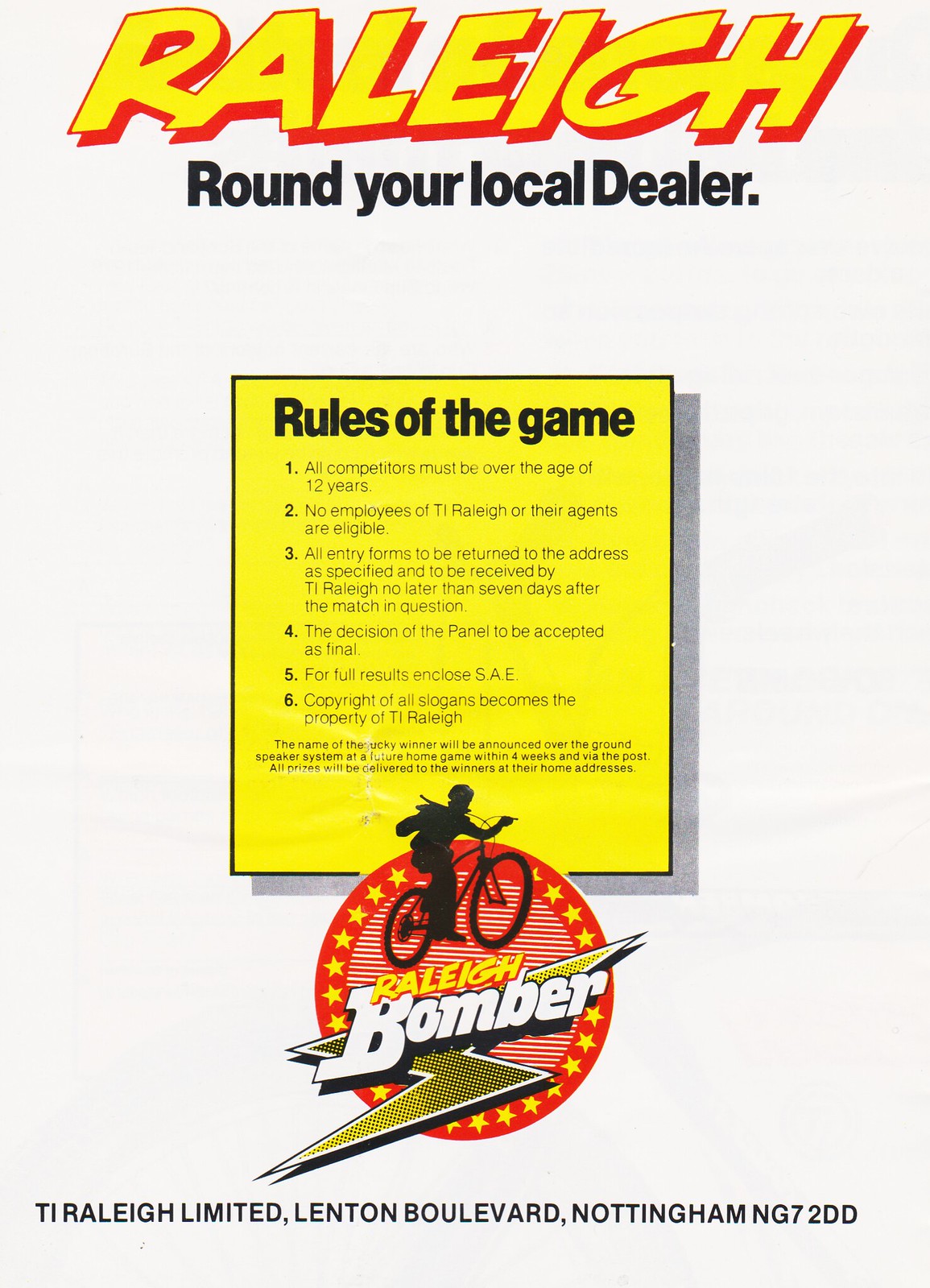The image is a detailed advertisement for the rules of a bicycling event titled "Raleigh Bomber" organized by T.I. Raleigh Limited. At the very top, in bright yellow letters, are the words “Raleigh” bordered in red, followed by “Round Your Local Dealer” in black font underneath. Centered on the large white board is a yellow rectangle labeled “Rules of the Game” in black text. 

The rules, written in small, detailed text, outline six key points:

1. All competitors must be over the age of 12.
2. Employees of T.I. Raleigh and their agents are not eligible to participate.
3. Entry forms must be returned to the specified address and received by T.I. Raleigh no later than seven days after the match in question.
4. The decision of the panel is final and must be accepted as such.
5. To get the full results, enclose a self-addressed envelope (S.A.E.).
6. The copyright of all slogans becomes the property of T.I. Raleigh.

Below these rules is a logo depicting a blacked-out figure riding a similarly blacked-out bicycle, jumping through a red circle adorned with yellow stars. Above this dynamic image, the event title "Raleigh Bomber" is prominently displayed in large white letters bordered in black. At the bottom, the text reads, “T.I. Raleigh Limited, Lenton Boulevard, Nottingham, NG7 2DD,” indicating the company’s address.